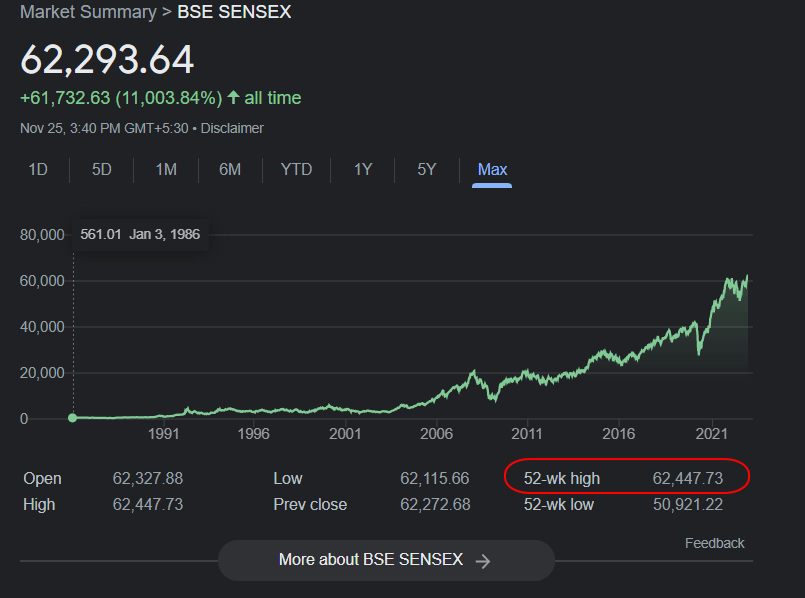A person is examining a market summary graph for a company, displayed on a dark-themed interface resembling Google Search. The user interface features a dark gray background with light gray accents, complemented by hints of light green and blue. In the top left corner, breadcrumb navigation traces the path: "Market Summary > BSE > SEN > SEX." Below this, a prominent figure, "62,293.64," captures attention, accompanied by numerous other numerical values.

The graph itself is accessed through multiple tabs, labeled: "1D," "5D," "1M," "6M," "YTD," "1Y," "5Y," and "Max," indicating various time frames from one day to several years. The "Max" tab is currently selected, presenting a comprehensive view of the data over the longest time span available. The x-axis of the graph denotes years, while the y-axis measures values in thousands. The graph depicts a positive trend, steadily ascending from left to right, albeit with some jagged fluctuations, resembling the gradual climb of a mountain.

Beneath the graph lies additional numerical data and descriptive information. At the bottom, a gray button labeled "More about BSE > SENSEX" features a right-facing arrow, inviting the user to explore further details.